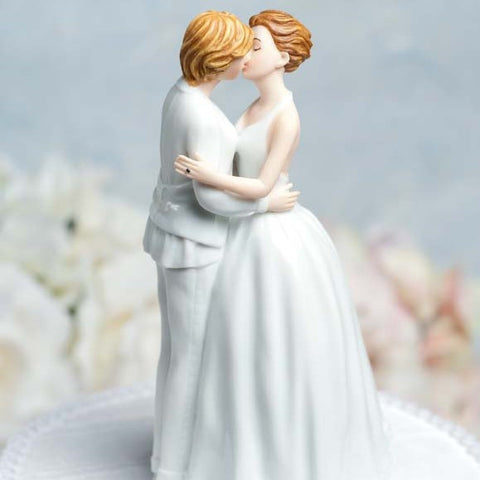In this photo of a wedding cake topper, the focus is on a pair of ceramic figures standing on a round, white base, which represents the top of the wedding cake. Against a bluish-white backdrop softened by out-of-focus white and pink flowers, the central figures share an affectionate kiss. On the left stands a figure with auburn, short hair, dressed in a white pantsuit that includes a jacket with sleeves reaching the wrists. Opposite, on the right, is a figure in a sleeveless halter-top white wedding gown with a full-length skirt, her shoulder-length brunette hair slicked back. She notably wears a black ring on her left hand. Both figures embrace each other warmly, creating an intimate and touching scene ideal for a wedding celebration.